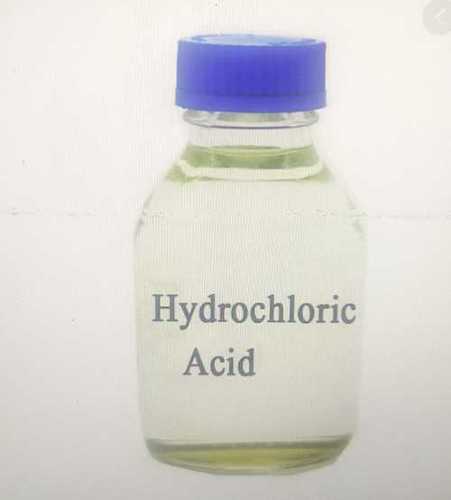The image depicts a small, clear glass bottle with a blue plastic screw-on cap, centrally dominating the scene. The background is an off-white color, creating a minimalistic and plain backdrop. The bottle, which appears to be made of either glass or plastic, contains a slightly yellowish, almost clear liquid. The label on the bottle prominently displays the term "Hydrochloric Acid" in black lettering, with "Hydrochloric" written on one line and "Acid" directly below it, although slightly indented to the left. There is a gray circular symbol to the top right of the label. The bottle is positioned on what seems to be a white table, further emphasizing its nondescriptive, generic nature, suitable for textbook illustration or simple product placement.